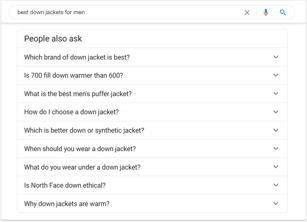This image is a cropped screenshot of Google search results for "best down jackets for men." The entire background is white. At the top of the image is the search bar, featuring rounded edges on both sides. Inside the search bar, in lowercase letters, is the query "best down jackets for men." To the right of the search text, there are three icons: an 'X,' a microphone, and a blue search icon.

Below the search bar, there is a thicker gray line, which appears somewhat like a shadow, marking the start of the main content section. This section begins with "People also ask," which is highlighted in black, sans-serif font, with the largest text size in the image. Each subsequent row features a slightly smaller font and contains frequently asked questions related to down jackets for men.

These questions include:
1. "Which brand of down jacket is best?"
2. "Is 700 fill down warmer than 600?"
3. "What is the best men's puffer jacket?"
4. "How do I choose a down jacket?"
5. "Which is better, down or synthetic jacket?"
6. "When should you wear a down jacket?"
7. "What do you wear under a down jacket?"
8. "Is North Face down ethical?"
9. "Why are down jackets warm?"

Each question is situated on its own row, each ending with a 'V' icon on the far right, indicating a drop-down menu for further details.

The section containing these questions is bordered by a thin gray outline, and each question row is separated by a thin gray line, adding structure to the layout. This minimalist design emphasizes the key search results without any additional distractions.